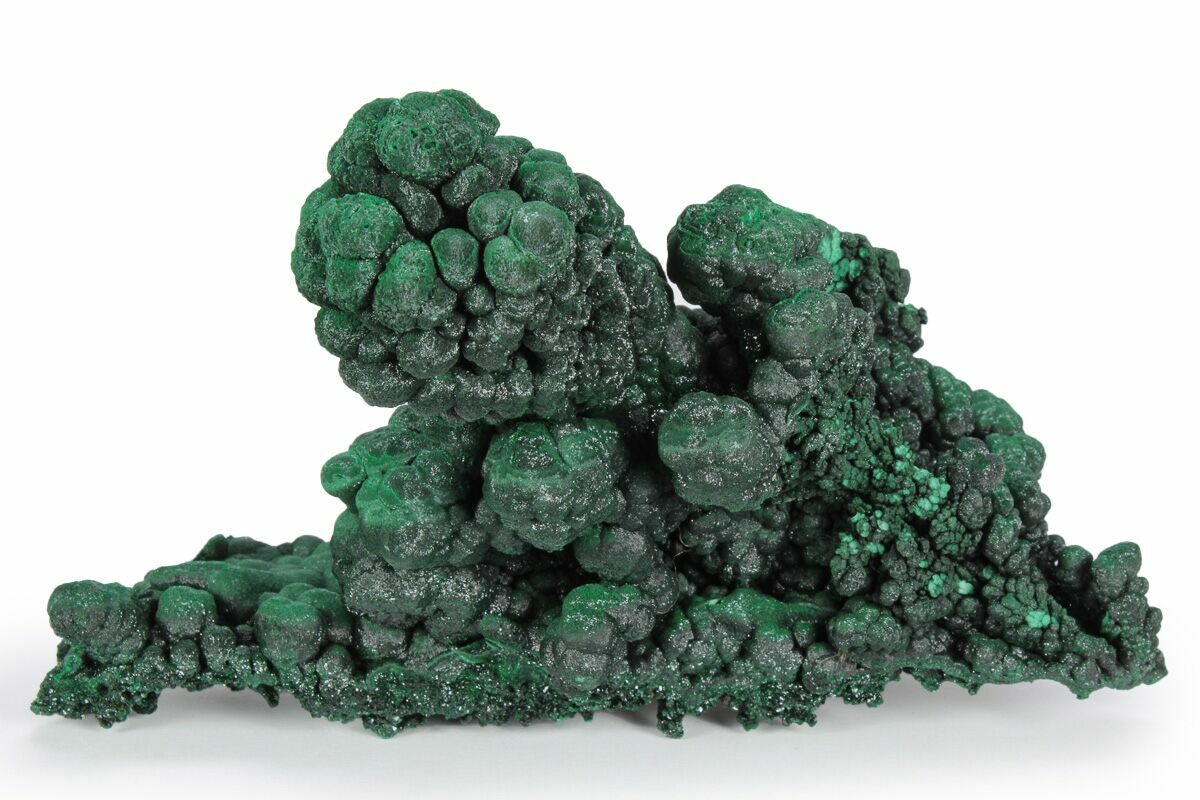The image showcases a dark green formation set against a plain white background. This striking piece resembles both a mineral and a coral, featuring a flat base with two prominent clusters that rise from it. The larger cluster on the right has a grenade-like appearance, while the smaller cluster on the left branches into many rounded, bubble-like growths. The overall texture of the sculpture is rough and jagged, reminiscent of moss-covered boulders or broccoli stalks. The formation features a spectrum of greens, including deep forest green, leaf green, and specks of mint green. Its organic, aged look suggests it might have been shaped and worn smooth by sea waves over time, giving it a textured, natural elegance that bridges the gap between rock and marine coral.